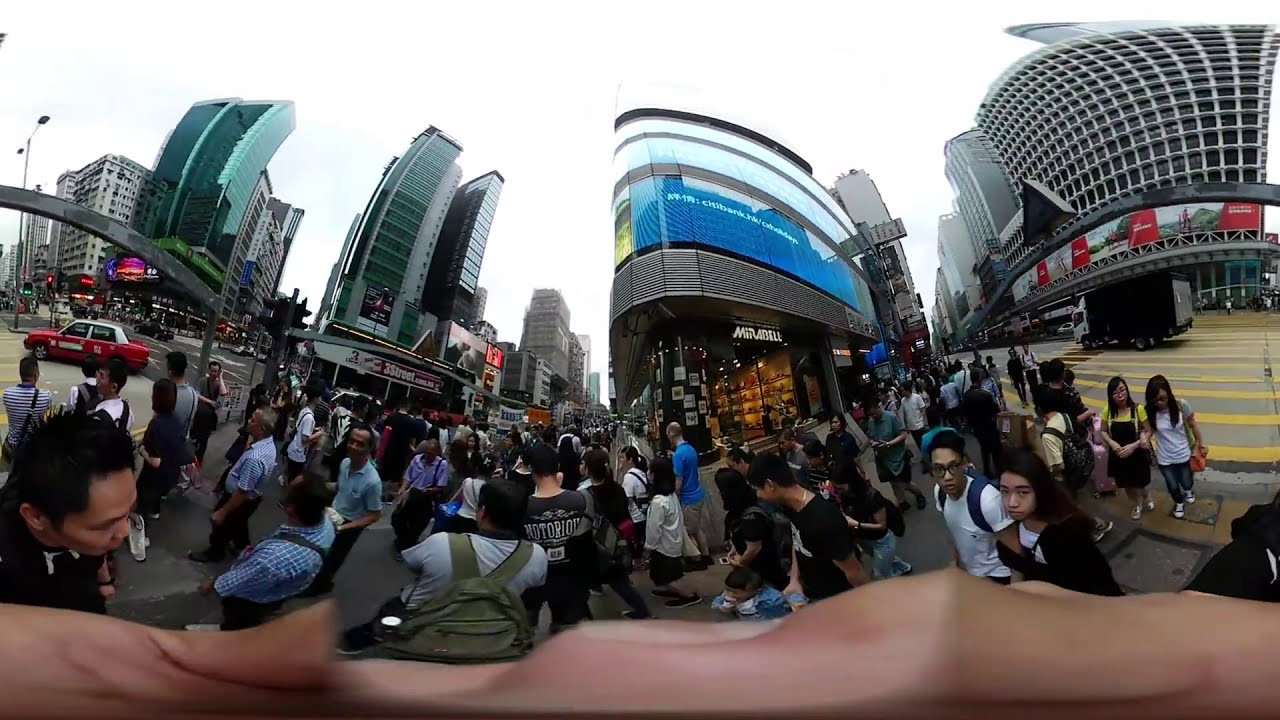The panoramic image depicts a bustling city street filled with a myriad of pedestrians. The scene is reminiscent of Tokyo or New York City's Times Square, characterized by an energetic, tourist-heavy atmosphere. On the left side, a distinctive red taxi with a white top stands out near a cluster of towering glass skyscrapers, alongside a smaller stone building adorned with mirrors. An overhead bridge or skywalk extends from one of the skyscrapers. The scene teems with people, some of them coming into clear focus, like a young boy in a white shirt with a blue backpack and spectacles, and a girl in a red shirt paired with a black jacket. In the bottom part of the image, there's a distorted view, perhaps of a hand, hinting at the panoramic nature of the photo. To the right, a colossal black-and-white semi-truck navigates the busy road. Amidst the vibrant cityscape featuring diverse colors—blue, black, white, teal, yellow, red, pink—various store signs and banners catch the eye, although they are largely indiscernible due to blurriness. A notable structure is an MGM building with a large banner. The sky above is a plain white, casting a bright light over the entire scene.